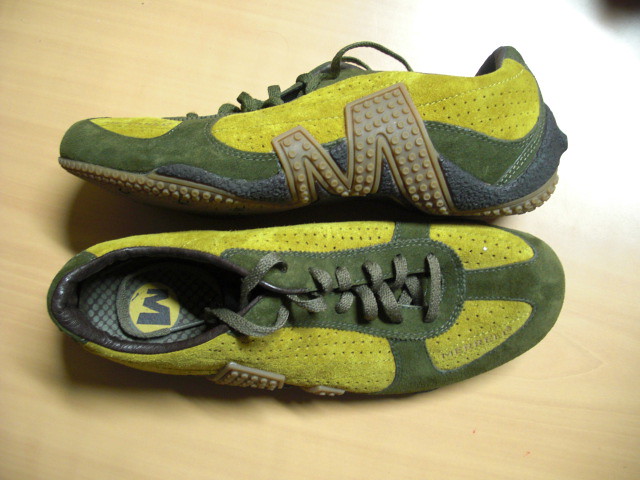A square image features a pair of sneakers positioned on a light brown wooden surface, possibly a table or floor. The sneakers showcase a mix of light green (sage or neon green) and dark green (hunter green) colors. The left shoe is tilted on its side, revealing a layered color pattern starting with a light green upper section, followed by a dark green middle, and a navy blue lower part above the textured brown sole. Green laces thread through the dark green eyelets. A prominent tan, rubber "M" logo with a nubby texture, reminiscent of Lego dots, is displayed on the side of the shoe. The right shoe lies flat, facing right, displaying similar detailing with green laces and dark green accents around the toe area. Light filters in from the upper right corner, highlighting the suede textures and extensive top stitching on the shoes. Inside, the insole features a dark "M" logo set within a greenish-yellow circle.